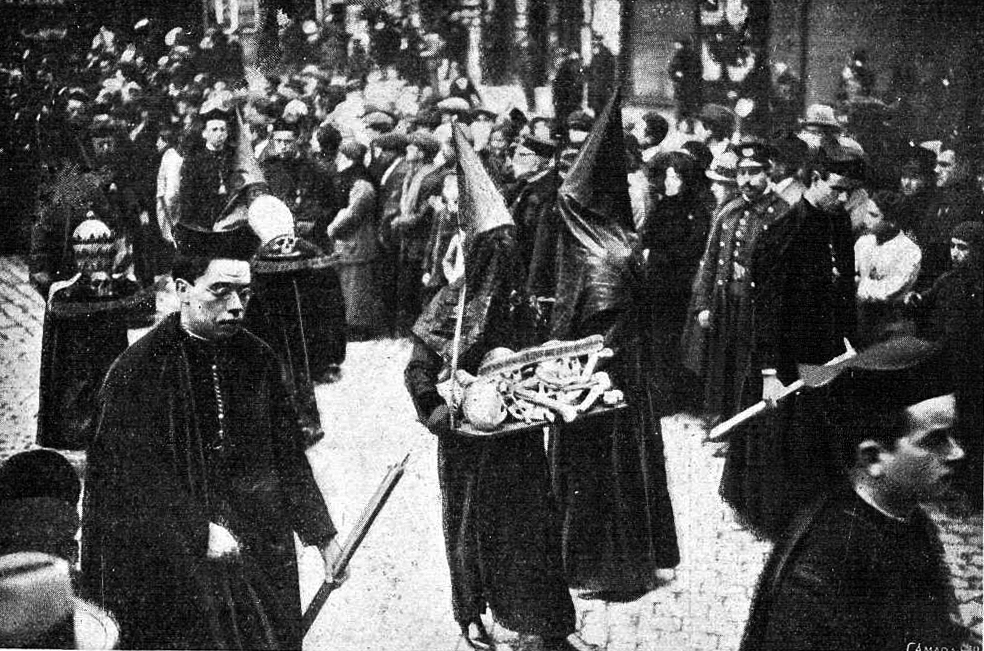The image is a black and white photograph, likely from the early 1900s, depicting a large crowd gathered on what appears to be a cobblestone street. Central to the scene are two individuals dressed in hooded black robes with large pointed hats, reminiscent of plague masks, creating an eerie and disturbing atmosphere. One of these figures is holding a tray laden with what appears to be human bones. This takes place during a religious procession, as evidenced by the presence of other individuals in ceremonial attire similar to priests, complete with crosses. The onlookers, which include a police officer, watch intently as the procession unfolds, adding to the gravity of the scene. This historical photo captures a significant and solemn moment, possibly in a European city such as Barcelona, with the detailed attire and the nature of the event suggesting a deep-rooted religious or cultural significance.